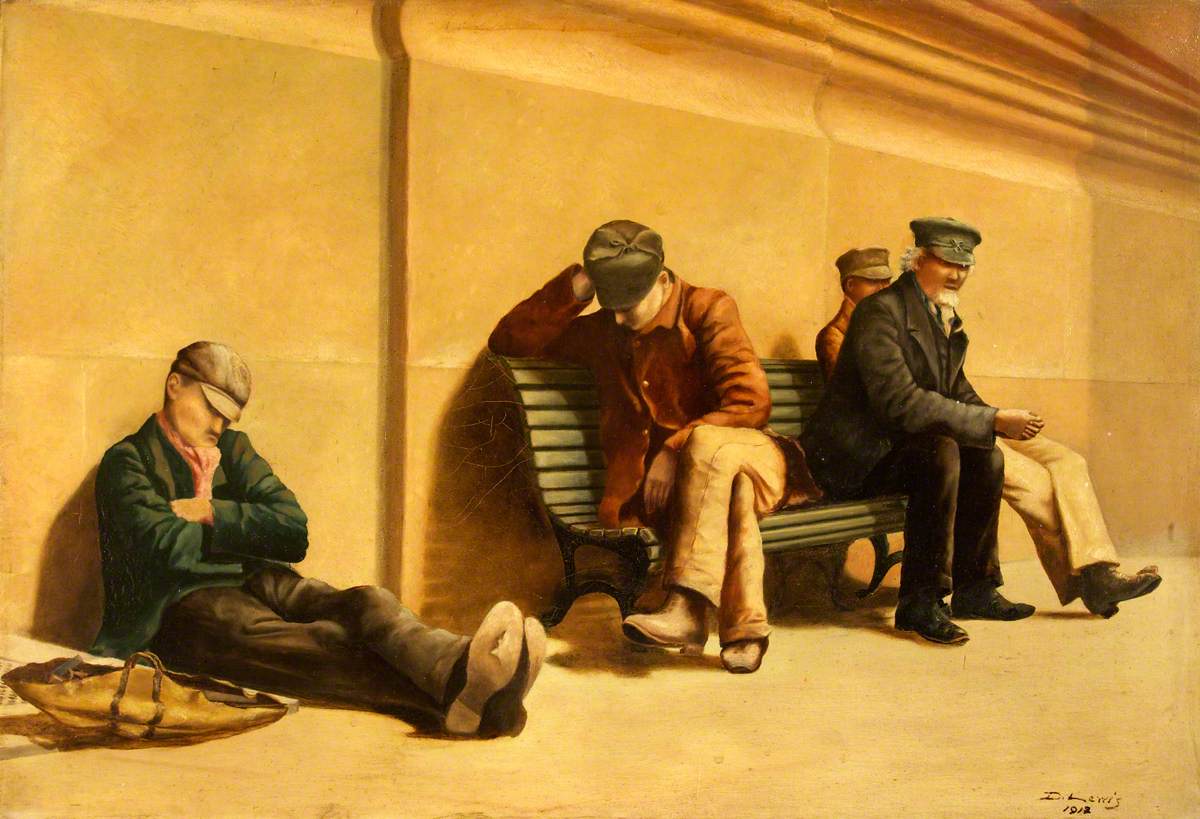This painting, marked with a small signature starting with an "I" and dated approximately 1912 or 1918 in the bottom right corner, exhibits a subtle yellowed or brown hue indicative of its age. The scene captures four men against a wall: three seated on a narrow-planked green park bench, and one lying on the ground with his legs crossed next to a paper bag with leather handles. The man on the ground is clad in a green long-sleeved coat, a brown cap with a bill, dark brown pants, and brown shoes—one of which has a noticeable mark on the sole.

On the bench, starting from left to right, the first man wears a reddish-brown coat, light brown pants, and brown shoes, and has his head resting on his right hand, appearing to doze off. Beside him is a man in a dark ensemble with a formal cap, resembling a train conductor's hat, adorned with an emblem. He sports a white beard and hair peeking out from under his cap. The last man, partially obscured by the conductor-like figure, dons a short rounded cap, a brown jacket, and light brown pants. The detailed sartorial choices and postures of the subjects add depth and character to this classic, early 20th-century artwork.